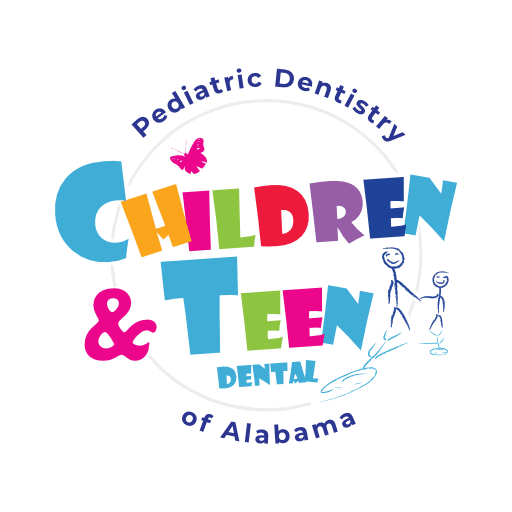The image is a square-format logo featuring a circular design on a white background. At the top of the circle, in dark blue text, it says "Pediatric Dentistry." Curving along the bottom arc, also in dark blue, are the words "of Alabama." Boldly written across the center and extending slightly outside the circle is "CHILDREN AND TEEN DENTAL" in playful, multicolored letters. Each letter in "CHILDREN" is a different vibrant color, with a dark pink butterfly serving as the dot over the 'I.' "TEEN" follows in similarly colorful typography, while "DENTAL" is in smaller, all-caps blue text. To the right of the circular logo, two stick figures are holding hands—an adult figure inside the circle and a smaller child figure outside. The stick figures are dark blue, with aqua blue shadow versions beside them. Both figures are smiling, adding to the playful and friendly appearance of the design.